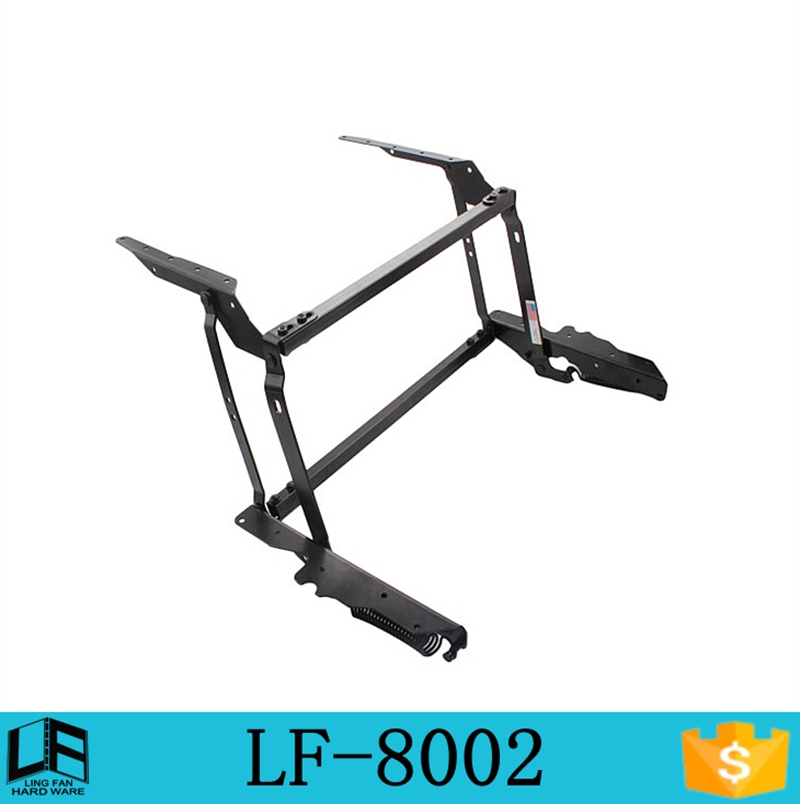The image features a unique metal structure prominently positioned at a diagonal angle against a white background, taking up most of the frame. The object, identified as a Coffee Table Lift Mechanism labeled LF-8002 by Lin Feng Hardware, is centrally placed and appears to be a stock image, possibly for website use. The mechanism, constructed of metal, includes springs, cross arms, and drilled holes on both sides designed for mounting a surface. A light blue banner at the bottom of the image displays the product name and company information. The colors in the image range from black, white, and light blue to accents of orange and yellow, enhancing the detailed view of this functional device meant to raise a coffee table surface closer to the user when in use.